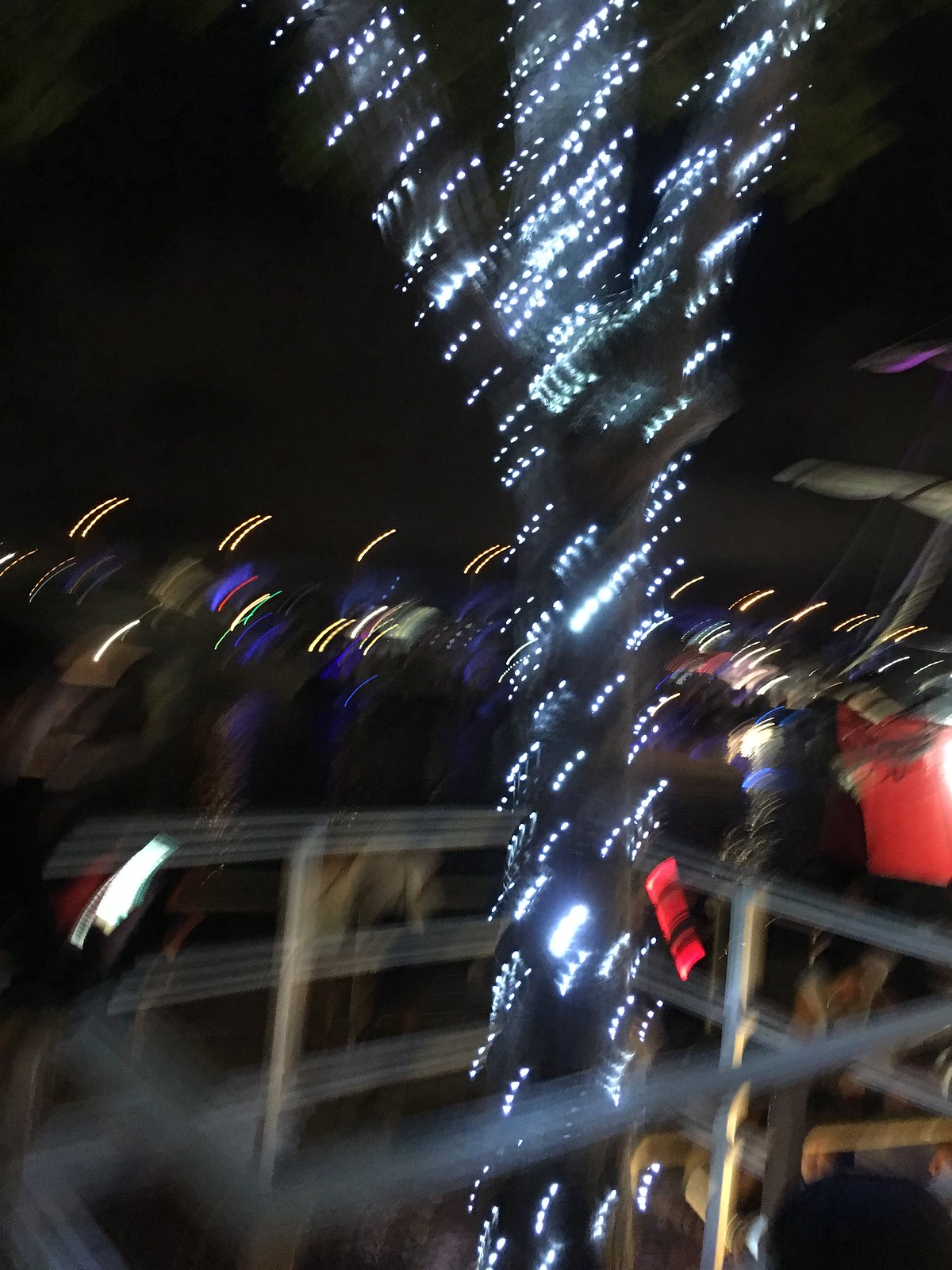The image appears to be set at night, characterized by a completely black sky. It is notably blurry, suggesting it was taken quickly or in motion. The focal point is a narrow tree adorned with white LED lights, possibly indicating a Christmas theme. The tree features three thin sub-trunks extending from the top. Surrounding the tree is a metal railing or fence, forming a square base. A crowd of indiscernible faces and movements gathers around the fenced area. Off to the right, there is a faint sliver of purple light, perhaps from a black light, hinting at a festive atmosphere. The backdrop and foreground suggest the setting is a party or gathering.